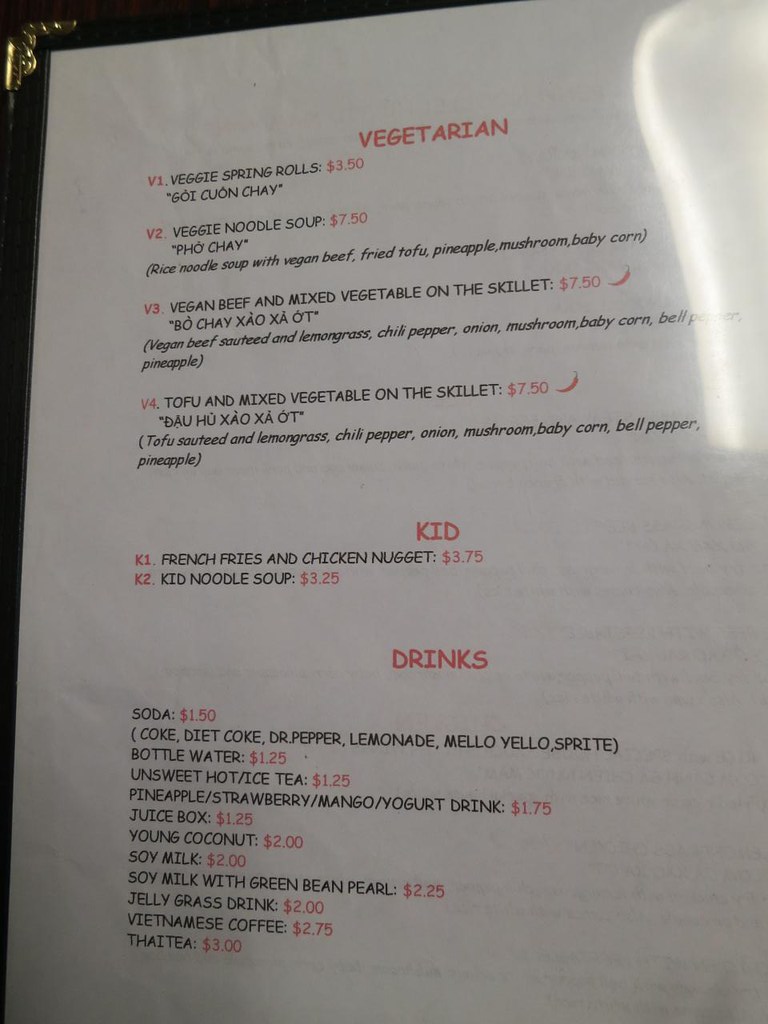The photograph features a laminated menu housed within a black, faux leather folder, complete with brass-colored decorative reinforcements on the top corners. The menu itself is protected by a clear plastic cover, allowing for easy cleaning in case of spills.

The menu is printed on white paper, utilizing a Comic Sans Serif font. Important headings and prices are highlighted in red, while the main body of text is in black. The section headers and meal descriptions are bilingual, with English accompanied by transliterated Vietnamese.

The Vegetarian section is prominently marked in red, with each item identified by a unique alphanumeric code. The first item, V1, is "Veggie Spring Rolls" priced at $3.50, listed with the Vietnamese equivalent "Chả Giò Chay." V2 features "Veggie Noodle Soup" (Phở Chay) at $7.50, described as containing rice noodles, vegan beef, fried tofu, pineapple, mushroom, and baby corn. V3, "Vegan Beef and Mixed Vegetables on the Skillet," also priced at $7.50, is marked with a red chili pepper, indicating it is a spicy dish. The Vietnamese translation follows as "Bò Chay Xào Sả Ớt." This dish includes vegan beef, lemongrass, chili pepper, onion, mushroom, baby corn, bell pepper, and pineapple. V4, similarly priced and marked as spicy, is "Tofu and Mixed Vegetables on the Skillet" ("Đậu Hũ Xào Rau Củ"), featuring tofu, an array of vegetables, and similar seasonings.

The next section caters to children (Kid's Menu), with K1 offering "French Fries and Chicken Nugget" at $3.75, and K2 presenting a "Kid Noodle Soup" for $3.25.

The Drinks section includes a variety of options such as soda (Coke, Diet Coke, Dr. Pepper, Lemonade, Mello Yello, Sprite), bottled water, hot or iced tea (unsweetened), yogurt drinks (pineapple, strawberry, or mango), juice boxes, young coconut, soy milk (regular and with green bean pearl), jelly grass drink, Vietnamese coffee, and Thai tea. Prices for the drinks are not detailed in the description.